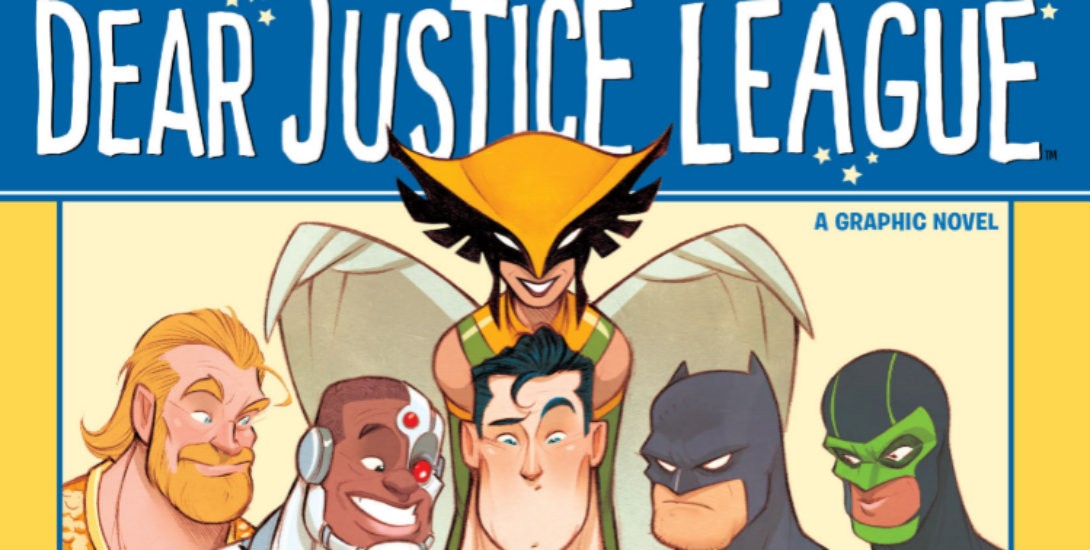The image shows the illustrated front cover of a graphic novel titled "Dear Justice League." It's only the top portion of the cover, framed by a blue rectangular box at the top where the title "Dear Justice League" appears in customized white, all-capital letters, set against a black field sprinkled with tiny, slightly yellow stars. Below the title, the text "a graphic novel" appears in smaller blue lettering on the right. The main section below features a muted light yellow background with six superheroes prominently displayed. From left to right, the characters include Aquaman, Cyborg, Superman (in the center), Batman, and an unidentified superhero with a green face mask. Behind them, partially obscured, stands a woman with wings dressed in a green and yellow outfit. The edges of the cover are partially cut off, which hides some details of the characters and their surroundings.